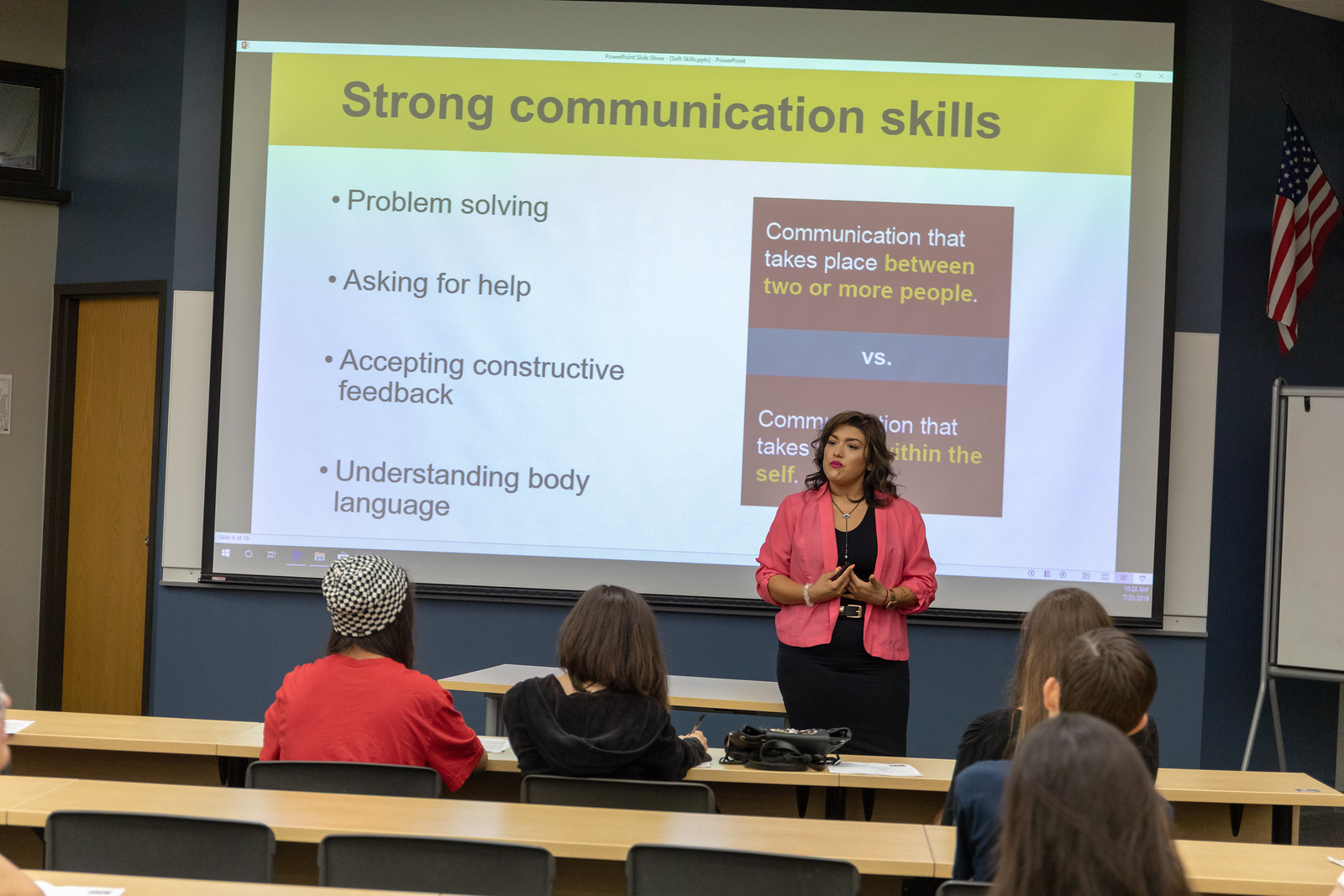In the image, a woman, likely a college professor, is giving a presentation in a classroom setting. She stands in front of a projector screen displaying a slideshow. She is dressed in a pink blazer over a black shirt with a black skirt, has shoulder-length black hair, and is wearing red lipstick. On the projector screen behind her is a slide titled "Strong Communication Skills" on a yellow banner. Below this, on a white background, are four bullet points: "Problem Solving," "Asking for Help," "Accepting Constructive Feedback," and "Understanding Body Language." Additionally, there is a red box with text, partially obscured by the woman's head, which reads "Communication that Takes Place Between Two or More People versus Communication that Takes Place Within the Self." In the classroom, five students are seated at long wooden tables, attentively watching the presentation. The room has a blue wall with a wooden door to the left and an American flag in the upper-right corner of the image.